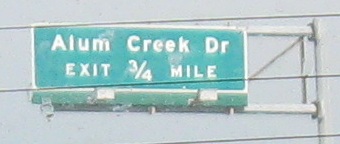In the image, a green highway sign for Alum Creek Drive can be faintly seen amidst a blurred backdrop. The sign, outlined in white, also indicates "Exit 3/4 Mile" below the main text. It is mounted on an off-white metal pole. There are three horizontal lines crossing the middle of the image, likely due to structural elements or artifacts, contributing to the overall lack of clarity in the photograph. The background is predominantly gray, and the edges of the metal pole exhibit digital artifacts, further emphasizing the image's out-of-focus quality.